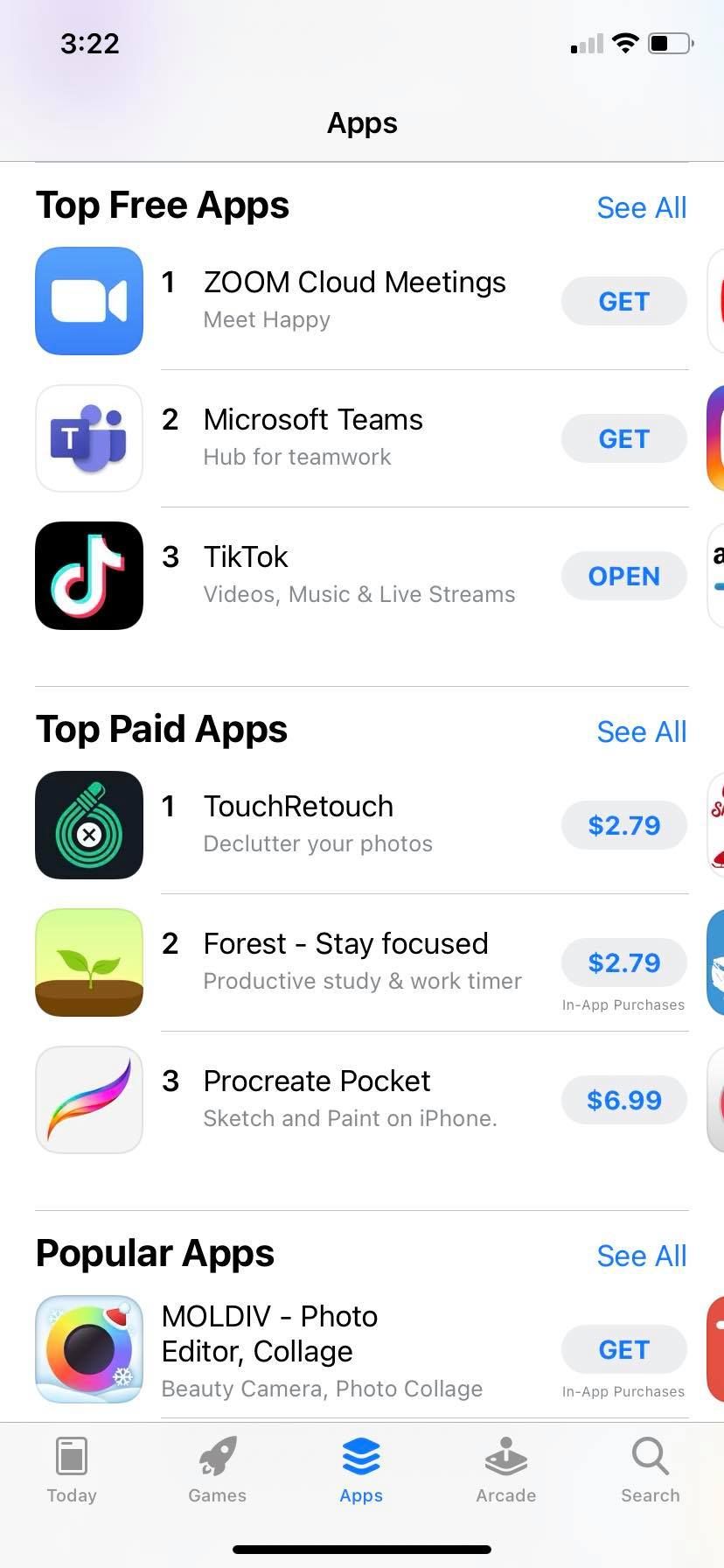**Caption:**

The screenshot captures the Apple Store interface on a mobile device, specifically showcasing the time of 3:22 in the upper left-hand corner. The precise time context of a.m. or p.m. remains unspecified. Noteworthy elements at the top of the screen include indicators for Wi-Fi strength, cellular signal strength, and battery level, which is approximately 40%.

This image reflects the typical aesthetic design and logo of the Apple Store app. Prominently displayed are various application icons and their respective details, outlining both top free and paid applications.

In the "Top Free Apps" section:

1. **Zoom Cloud Meetings** – Described as "Meet happy"
2. **Microsoft Teams** – Referred to as a "Hub for teamwork"
3. **TikTok** – Characterized by "Videos, music, and live streams"

Following the free apps, the "Top Paid Apps" section lists:

1. **TouchRetouch** – "Declutter your photos" priced at $2.79
2. **Forest - Stay focused** – "Productive study and work timer" costing $2.79 with in-app purchases
3. **Procreate Pocket** – "Sketch and paint on iPhone" available for $6.99